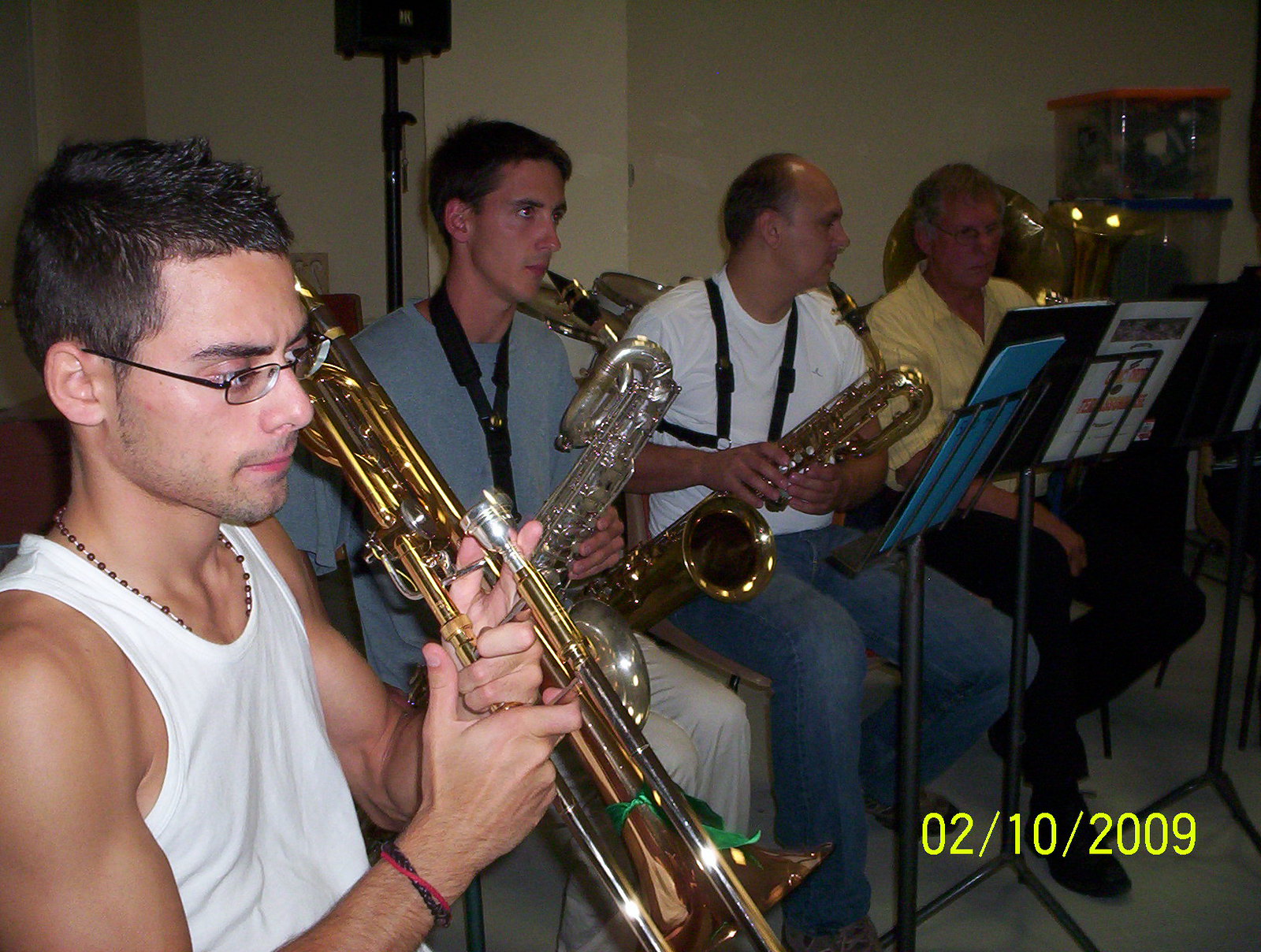This photograph, dated February 10th, 2009, captures four men seated in a rough J-shaped formation, each holding a large musical instrument, with a focus towards the right side of the image, possibly towards sheet music. The first man, nearest to the camera, is wearing a white tank top and small glasses while holding a trombone. Next to him, a man in a blue shirt and white pants grips a saxophone. The third individual, clad in a white shirt and jeans, also holds a saxophone. Finally, the man furthest from the camera, appearing to be in his 60s and dressed in a yellow button-up shirt and black pants, seems engaged with sheet music placed in front of him, beside a small tuba-like instrument. The informal attire of jeans and t-shirts suggests a casual setting, possibly a practice session. The scene is indoors, with a plastic container visible in the background. The exact date "02-10-2009" is noted in yellow font in the bottom right corner of the image.